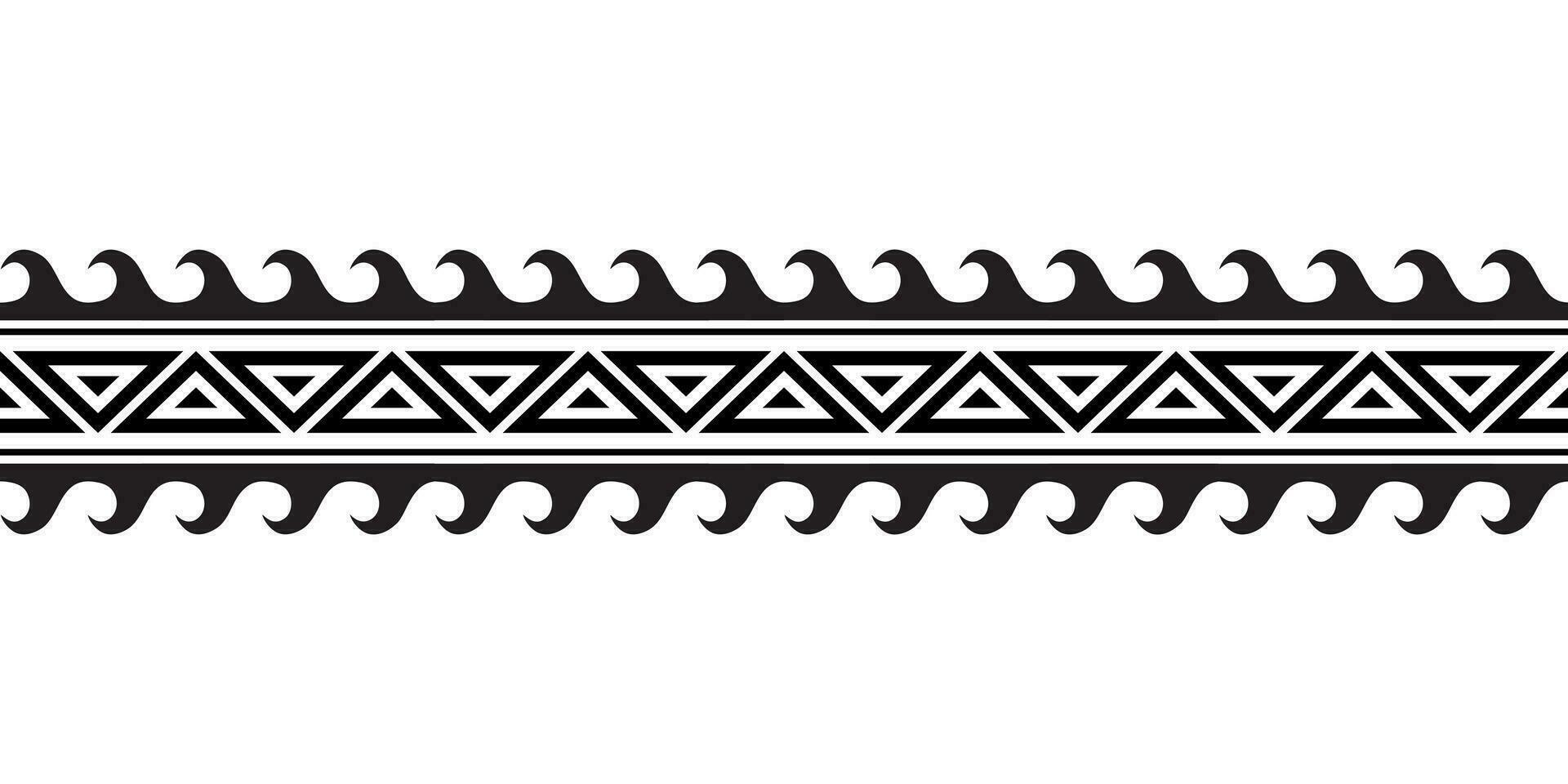The black and white geometric design appears to be inspired by Polynesian motifs, characterized by its intricate and repeating patterns. Dominating the center, a series of alternating triangles create a striking visual rhythm, with each sequence involving three distinct layers. The innermost triangle is black, followed by a white middle layer that essentially outlines the inner triangle, and an outer black layer. This pattern of alternating triangles, pointing up and down, repeats across the wide expanse of the image.

Flanking these triangular motifs are delicate white borders that separate them from adjacent elements. Along both the top and bottom edges of the design, black lines serve as the base for wave-like patterns that resemble ocean waves or barbs. These curved wave shapes extend toward the center, creating a dynamic framing effect on the design. The peaks of these waves typically point to the left, while the curves descend to the right before flipping upward again.

The entire image rests on a white background, emphasizing the stark contrast of the black geometric and wave patterns. The overall effect is reminiscent of traditional Polynesian art, which can be utilized in various applications such as tattoos or decorative borders on paper.